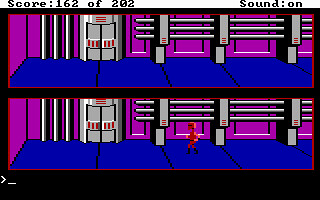This image appears to be a screen capture from a vintage or retro-style platform game, characterized by its low resolution and small scale, reminiscent of early handheld gaming devices. The entire background is black while the platforms themselves exhibit a distinct color scheme: the background within each platform is pink, the floor is blue, and there are various grey shapes resembling horizontal pipes and a doorway located on the left side. The game screen is divided into two horizontal rows or levels, with one positioned above the other. At the very top of the image, the text reads "Score 162 of 202." In the top right corner, the words "STOUND ON" are displayed. In the bottom section of the image, a red and orange figure can be seen slightly to the right of the center, likely representing a character or player avatar navigating through the game.